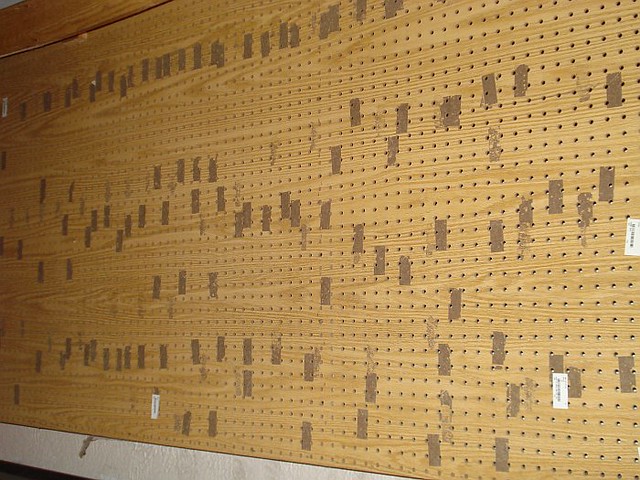The image depicts a large, light wood pegboard featuring a grid of numerous evenly spaced small circular holes. The board is marred by various dark brown adhesive residue spots, indicating previous attachments of tape or stickers that have since been removed. There are also three to four white labels with blurry, black text that appear to be either barcodes or simple writing, positioned mostly vertically. The board's natural wood grain runs horizontally, adding texture to its surface. Situated in a mostly empty setting, the pegboard is flanked at the bottom by a gray strip, possibly part of a white wall or frame, and at the top by another section of wooden framing. The overall image captures the worn, utilitarian character of the pegboard, emphasizing its many uses over time.